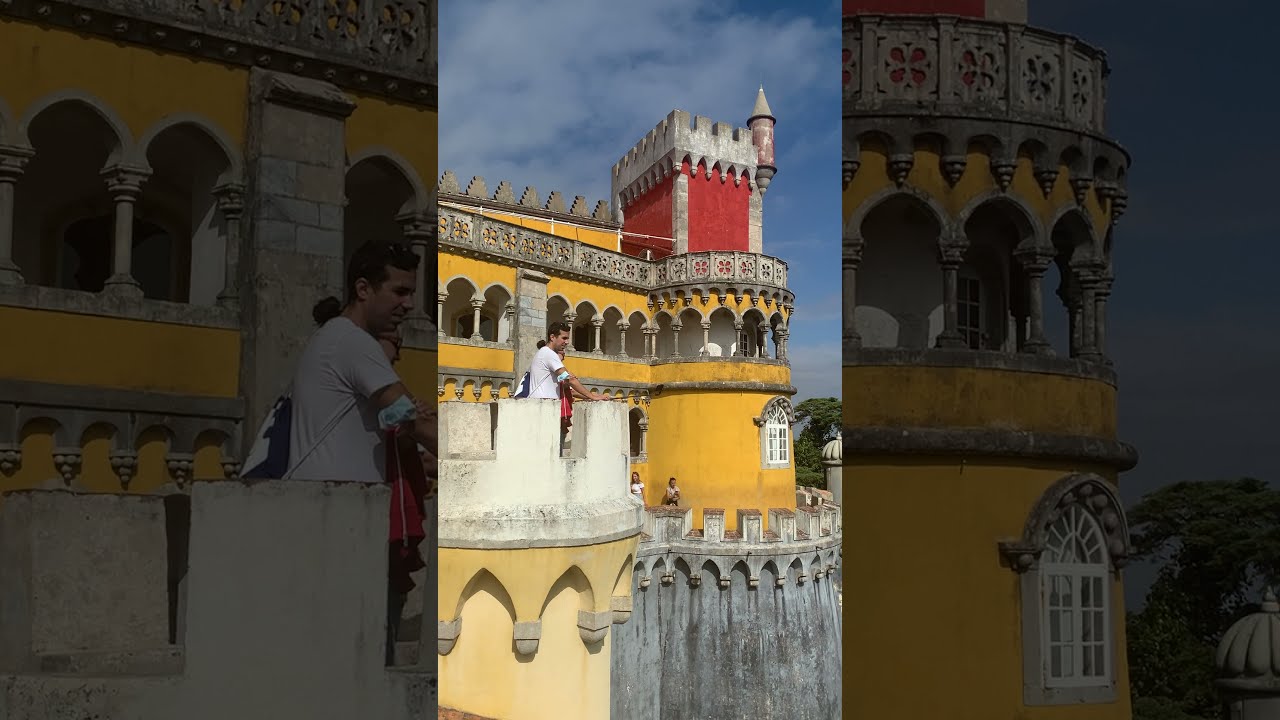In this image, we see a beautiful, ornate castle that exhibits a mix of vibrant colors and intricate architectural details. The castle features various turrets, some painted in an orangish-yellow hue, while the tallest turret in the background is prominently painted red and capped with a dome that evokes the shape of a tiny rocket. The turret in the lower left corner, on which a couple of people are standing, is tan-colored and has a parapet design reminiscent of a chess castle piece. The scene is set outdoors in the middle of the day under a blue sky with sparse, wispy white clouds.

The people at the top of the tan turret are facing to the left. One of them, a man with darker skin, possibly of Indian descent, is wearing a white t-shirt. Behind him, a woman with her hair in a bun is faintly visible, dressed in something red. The castle itself showcases a blend of yellow, white, gray, red, and gold colors, with elaborate stone carvings and architectural grandeur. The overall picture captures an ancient, antique charm, highlighting the castle's historical and aesthetic significance.